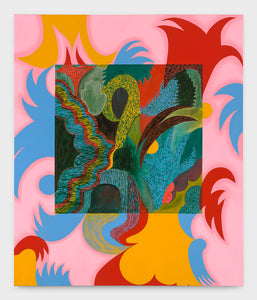This image showcases an intriguing piece of modern abstract art against a white background, potentially a product photo. The artwork appears as a vibrant, abstract painting framed within another painting, creating a layered, dynamic effect. 

At the heart of the piece is a central square, rich in deep, darker hues with intricate, jagged swirls and lines. These central elements evoke the essence of a tropical forest, featuring sharp, leaf-like patterns in green and brown, alongside zigzagging red swirls reminiscent of a red leopard print. A prominent yellow swirl with green dots resembles a coiled snake, while a multicolored zigzag pattern rimmed in red with blue, yellow, and red gradients adds a rainbow-like flourish.

Surrounding this central square is an outer frame brimming with pastel and brighter colors. Here, leaf-like swirls and patterns appear in dark red, light blue, yellow, and pink, sometimes blending into each other for a soft, harmonious effect. The entire composition exudes vibrancy and intrigue, punctuated with a hint of orange glow, yet maintaining a non-threatening, appealing allure. This complex modern pop art piece beautifully combines abstract motifs and a colorful palette, exemplifying contemporary artistic creativity.